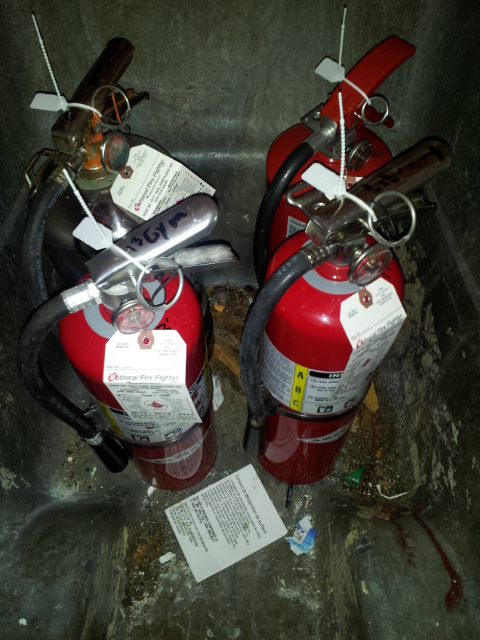The photograph, displayed in portrait orientation and taken from an elevated perspective, captures a group of four fire extinguishers arranged in a metal enclosure, possibly a crate. The interior appears worn and somewhat dirty, with noticeable rust spots along the metal flooring and walls. A white label with black writing lies on the floor.

The fire extinguishers are set in two rows: two in the front and two in the back, all facing the same direction as evidenced by the alignment of their handles. Three of the extinguishers are red, while the one in the top left corner is black. Each extinguisher is equipped with a white tag featuring written information and a black hose. The handles on the front row extinguishers are metallic silver, whereas the back row has one metallic silver handle and one red handle. Additionally, each handle assembly includes a zip-tie mechanism typical for safety seals. The overall ambiance of the scene is somewhat dark and gritty due to the lighting and shading in the photograph.